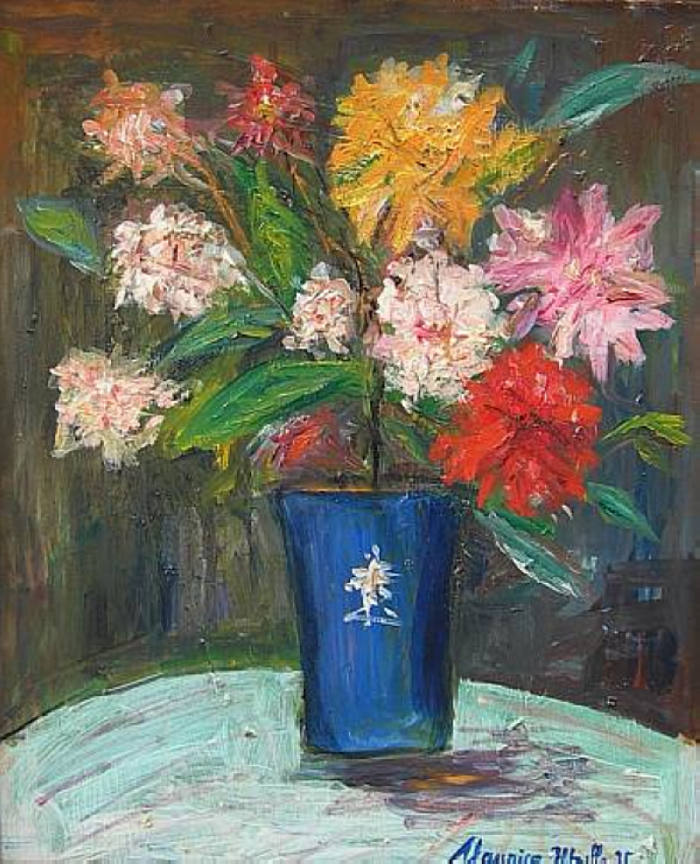The image depicts a flower bouquet in a blue, cobalt-colored vase, adorned with a white floral design in its center. This vase is placed on a distinctive turquoise table with gray swirling patterns, alongside a visible purple shadow marking the vase's placement. The substantial bouquet, consisting of approximately ten flowers, showcases a vivid range of colors including red, orange, light pink, and pink, complemented by green leaves. The background is a textured dark gray wall, infused with hints of green and blue. The painting features noticeable brushstrokes and is signed illegibly at the bottom. Overall, the scene is a vibrant yet rustic composition, suggesting the work of a budding artist, and would be a fitting decoration in a cozy home.